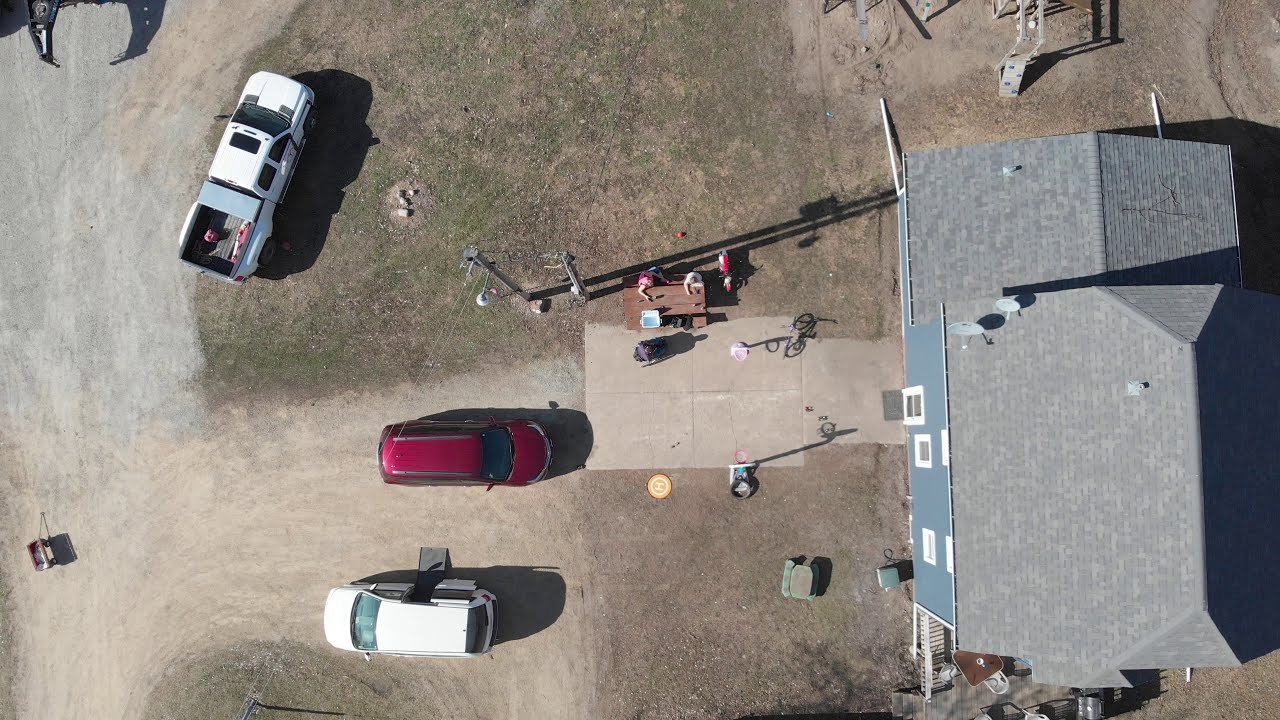This is a detailed aerial drone photo of a modest rural residence, capturing a range of notable features. The focal point of the image is a two-story house with a gray roof and sky-blue walls, adorned with white trim. Three white-framed windows are visible on the side of the house. Adjacent to the house are scattered metal objects, possibly poles or other materials, though their specifics are indistinct.

Three vehicles are prominently featured on the property, parked near a dusty, unpaved driveway with sparse, dying grass. At the bottom of the image, a white vehicle, possibly a minivan, has its door open, facing the left side of the image. Towards the middle of the image, a red sedan or SUV is stationed near a concrete or asphalt area leading to the house. In the upper left section, a white truck is parked in a grassy area that appears predominantly dead.

The house's entrance is towards the center-right of the image, where a small patio area is visible. On this patio, about three people are seated at a picnic bench near the concrete pad in front of the house. Behind them, a metal fence is evident, alongside some structures that might include electric poles or lampposts.

Overall, this detailed photograph captures a tranquil scene, reflecting the simplicity and rustic charm of its rural setting.